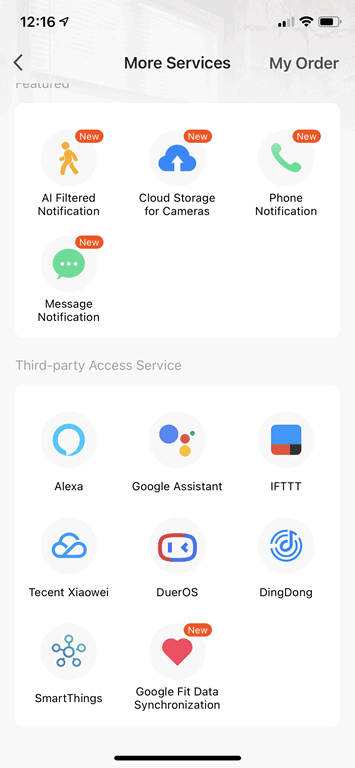The screenshot displays a user interface with several icons and text. Starting from the top right, we see a battery icon, followed by a full-bar Wi-Fi symbol, and a phone signal strength icon with two out of four bars. The current time, shown on the top left, is 12:16. Centered at the top in bold text is "Detects more services," with "More" to its right and "My Order" to the left, alongside a black arrow pointing left.

Below this, within a white box area, there are four icons arranged in two rows. In the first row, from left to right, are:
1. "Filter Notification"
2. "Cloud Storage for Cameras"
3. "Phone Notification"

In the second row, there is only one icon: "Message Notification."

Further down, the text "Third Party Access Service" is displayed above another white box area that contains eight icons arranged in three rows. In the first row, we see:
1. "Alexa"
2. "Google Assistant"
3. "IFTTT"

In the second row, from left to right, we have:
1. "10 Percent"
2. "Your OS"
3. "Ding Dong"

In the last row, there are two icons:
1. "SmartThings" on the far left
2. "Google Fit Data Synchronization" on the right.

Each element is clearly laid out, making the interface organized and user-friendly.